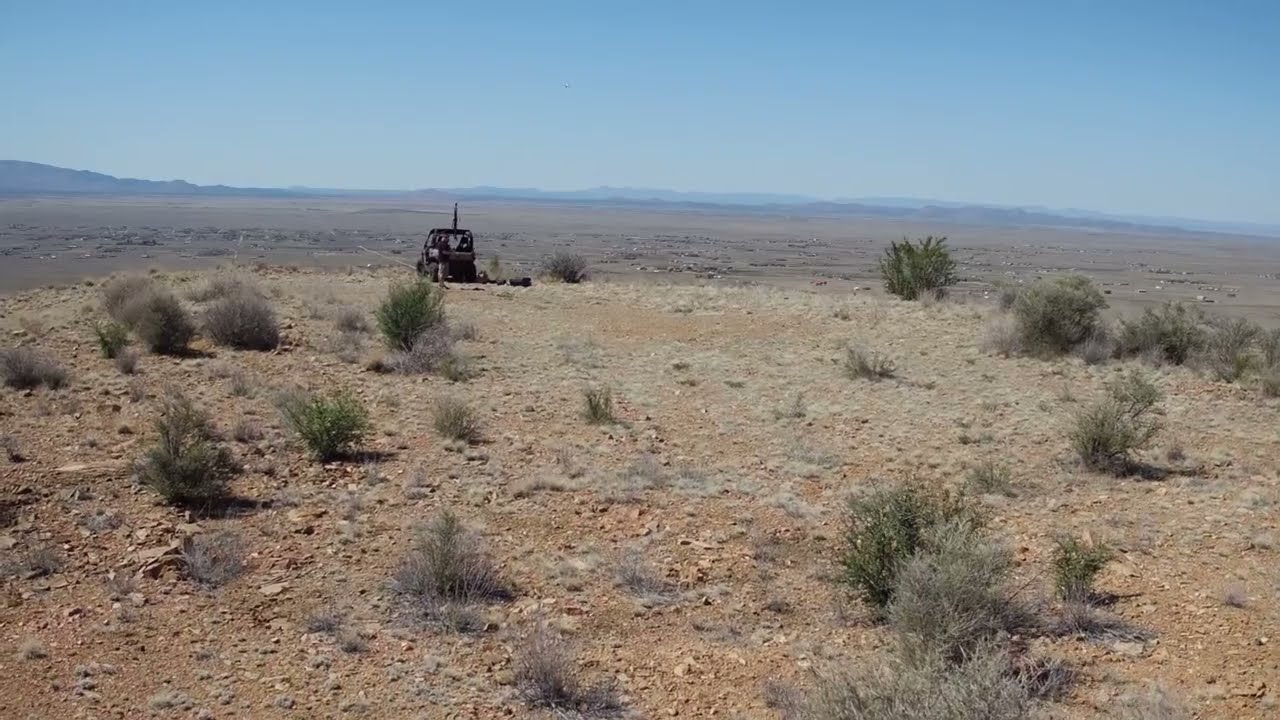The photograph captures a desolate desert landscape dominated by a vast expanse of dirt and rocks, punctuated by sporadic shrubs and dried-out tumbleweeds. The terrain, predominantly brown, extends endlessly, revealing a flat, arid surface with occasional stones and very dry, small patches of green vegetation. Toward the left side of the image, slightly above the middle, lies the rusted remnant of what seems to be a broken-down vehicle, probably the rear end of a truck, with an antenna protruding from it, further emphasizing the abandoned feel of the scene. In the background, subtle silhouettes of low-lying hills and a small mountain range faintly emerge on the horizon. The sky above is an unblemished gradient of blue, transitioning from a lighter hue near the horizon to a deeper azure at the top, underscoring the brightness of the sunny day. No clouds mar the clear sky, and the overall palette consists of earthy tones—browns, greens, grays, blues, and blacks, capturing the essence of this stark, uninhabited desert expanse.